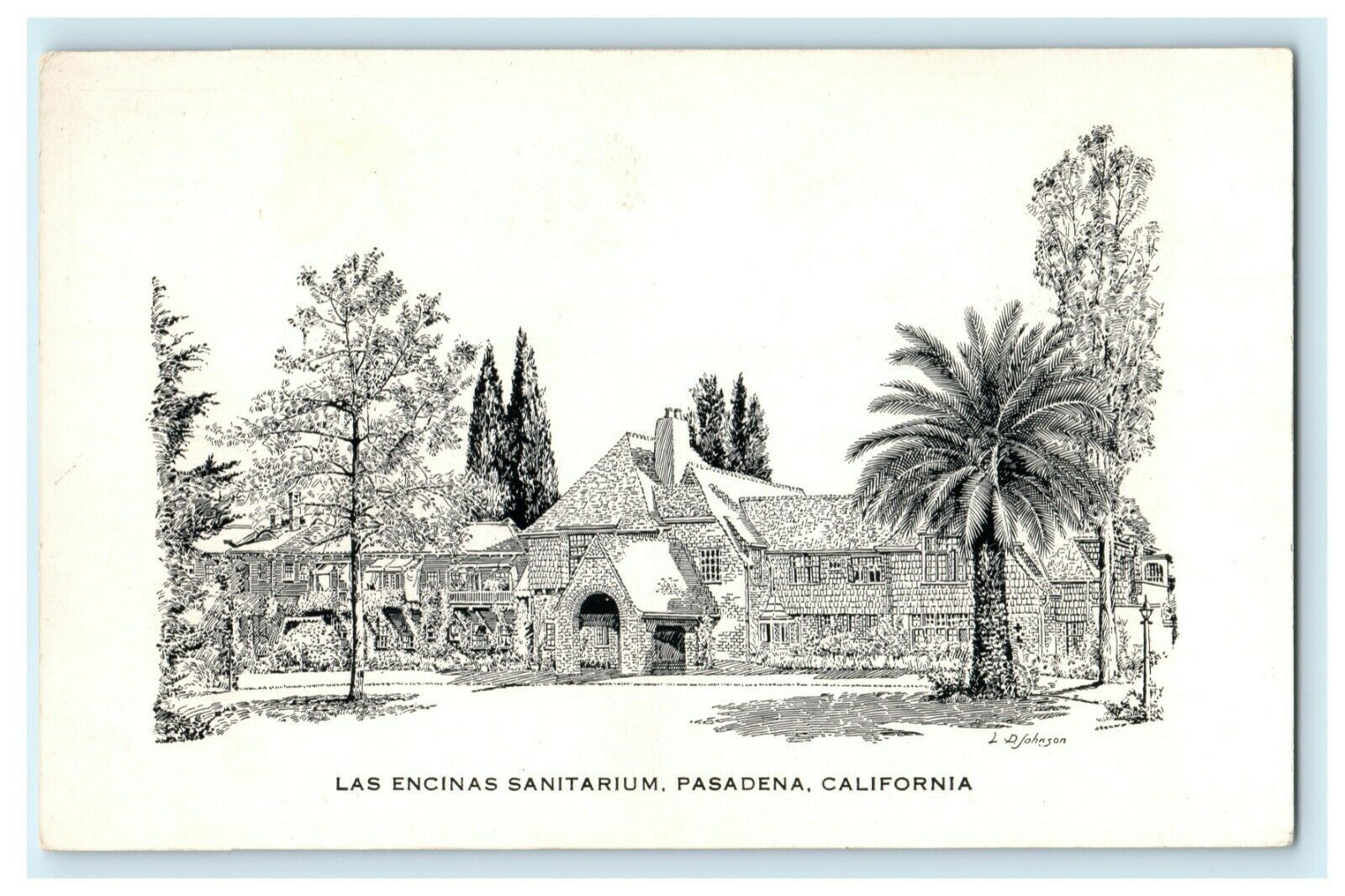This detailed pen and ink drawing presents a finely etched depiction of Las Encinas Sanitarium in Pasadena, California. The black and white artwork captures a series of interconnected buildings, primarily showcasing a large, two-story structure with numerous sections extending to the right and left. Prominent architectural features include a sheltered drive-through area in the front and windows with bar-like divisions. Nestled amidst a diverse array of lush trees, including tall palm trees, deciduous, and pine trees, the intricate etching vividly portrays the verdant surroundings. The foreground reveals a small mailbox located in the lower right-hand corner, while the background showcases more trees emerging above the buildings. The sky is rendered as the blank, white page of the paper, emphasizing the contrast between the dark ink and the white space. At the bottom of the drawing, the title "Las Encinas Sanitarium, Pasadena, California" is inscribed, accompanied by the artist's name.